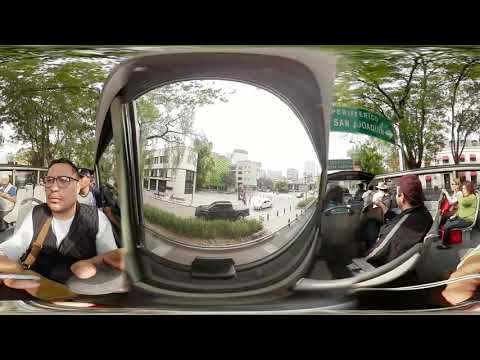This image, possibly taken through a round window or a mirror, features a detailed scene both inside and outside. On the left side, there is a man seated in a vehicle. He has short brown or black hair, wears glasses with black frames and clear lenses, and is dressed in a white long-sleeve shirt under a sweater vest, with a strap around his right shoulder. His hands are positioned in front of him. To the right, several people are seated, possibly on a ride, and positioned under a green street sign displaying text, possibly "San Joaquin." The setting outside the window or mirror includes a street bordered by small shrubs, with tall trees on both sides and several white buildings in the background. On the street are two vehicles: a black truck and a white BW. The photograph is slightly skewed, which adds to the complexity of the scene. The overall composition captures a blend of human activity within a vehicle against the urban backdrop of a city.